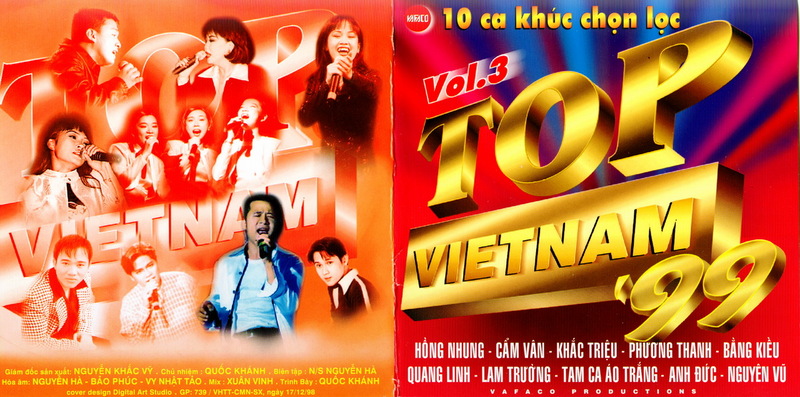The image resembles the cover and back of a CD case. It is divided into two panels, indicating the front and back. The left panel features the title "Top Vietnam" at the top, with three rows of people singing into microphones. The top row showcases a mixed group of singers, the middle row consists mostly of women, and the bottom row displays a group of men or young men. Yellow Vietnamese names are listed at the bottom. The image has a vintage, somewhat 3D appearance with a red color shift, although one individual in the bottom row is in full color.

The right panel features a red and blue background with the title "Volume 3 Top Vietnam-99" in gold letters at the top, and "Top Vietnam" in red letters. At the bottom, various Vietnamese names are listed in white letters.